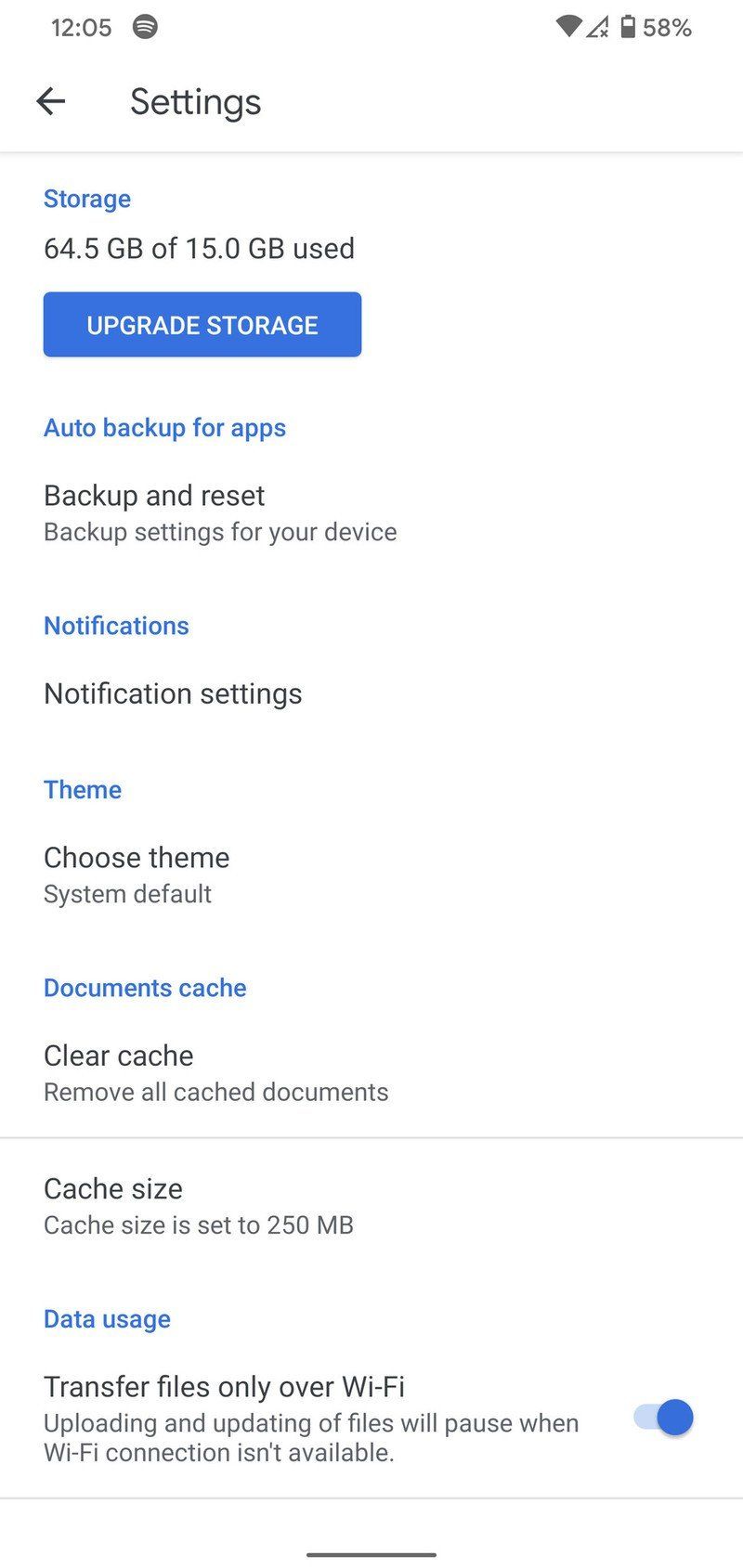Screenshot of Phone Settings Menu

This screenshot depicts a phone's settings interface captured at 12:05. Located in the upper portion of the image, the status bar shows active Wi-Fi and a battery level at 58%. A triangle symbol is also present, though its meaning is unclear.

Below the status bar, a horizontal grey bar contains a left-arrow icon and a text label reading "Settings." The primary settings list begins with a blue-highlighted "Storage" option, accompanied by the information "64.5 GB of 150.0 GB used" in black text. A blue button underneath, labeled "Upgrade Storage" in white font, suggests options for increasing storage capacity.

The next setting, "Auto Backup for Apps," is in blue, while "Backup and Reset" is in black with a description, "Backup settings for your device." Following this, "Notifications" in blue is paired with "Notification Settings" in black.

The section for "Theme" is listed next, with "Choose Theme" in black, displaying options such as "System Default," "Parallel," and "Current Theme." Further down is "Documents Cache" in blue and "Clear Cache" in black, with a description that indicates this option will "Remove all cached documents."

A grey horizontal line separates this from the next section that specifies the cache size, set to "250 MB." The last item in the list is "Data Usage" in blue.